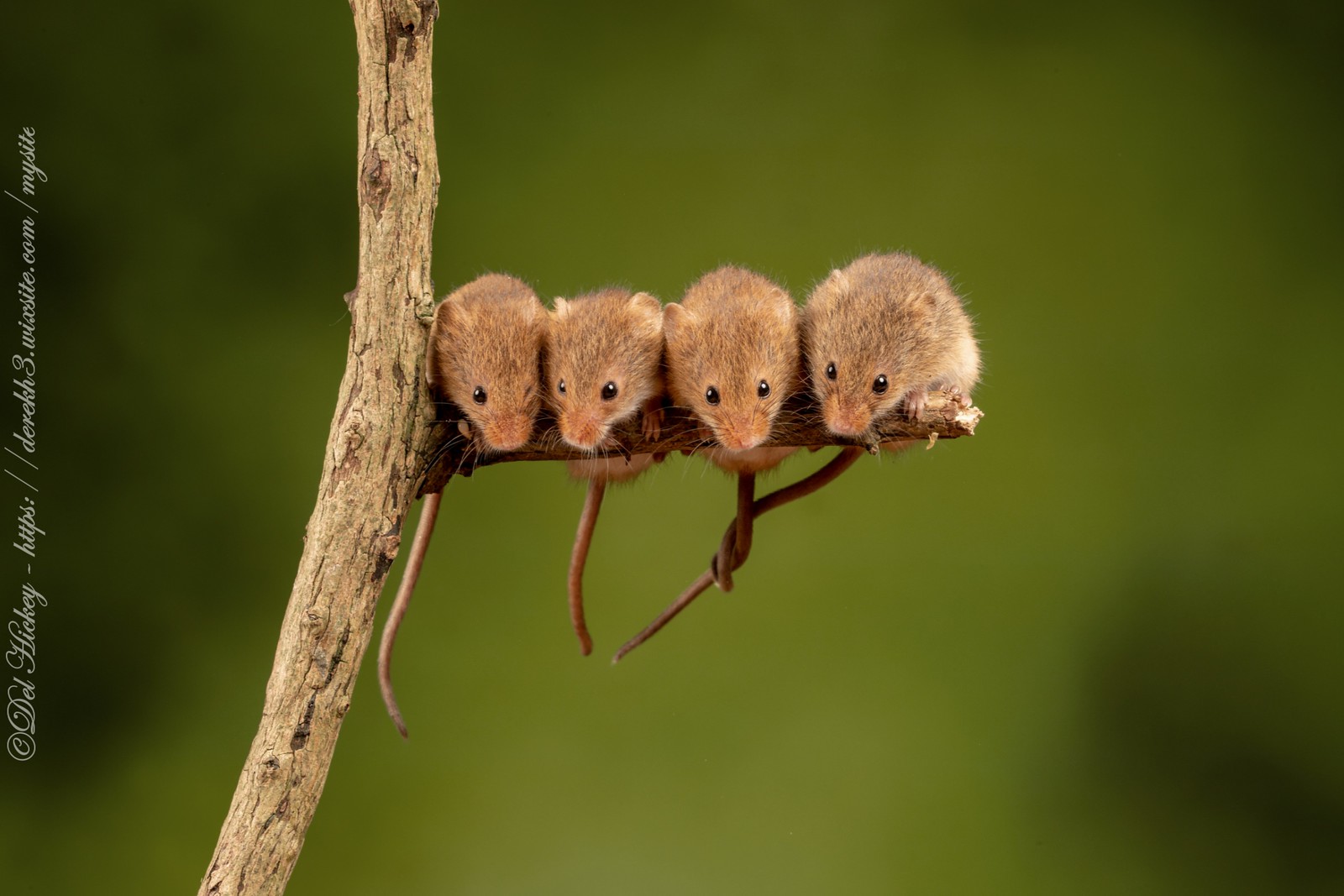This close-up photograph shows four light brown mice clinging to a small, brown branch. The branch itself has a light tan hue with darker brown knots, and its peeling, cracked bark is clearly visible. Captured in a front view, the mice each feature two little black beady eyes, slightly visible ears, and chocolate brown noses. Their fur, which extends from their noses toward their crowns, gives them a round appearance. The rightmost two mice have their tails intertwined, while two other tails dangle freely. The green background is heavily blurred, suggesting a forest setting. On the left side of the image, cursive text reads "copyright delhickeyhttp-derrick3.weasight.com/mysight." This text might be indicative of the photograph's copyright information.